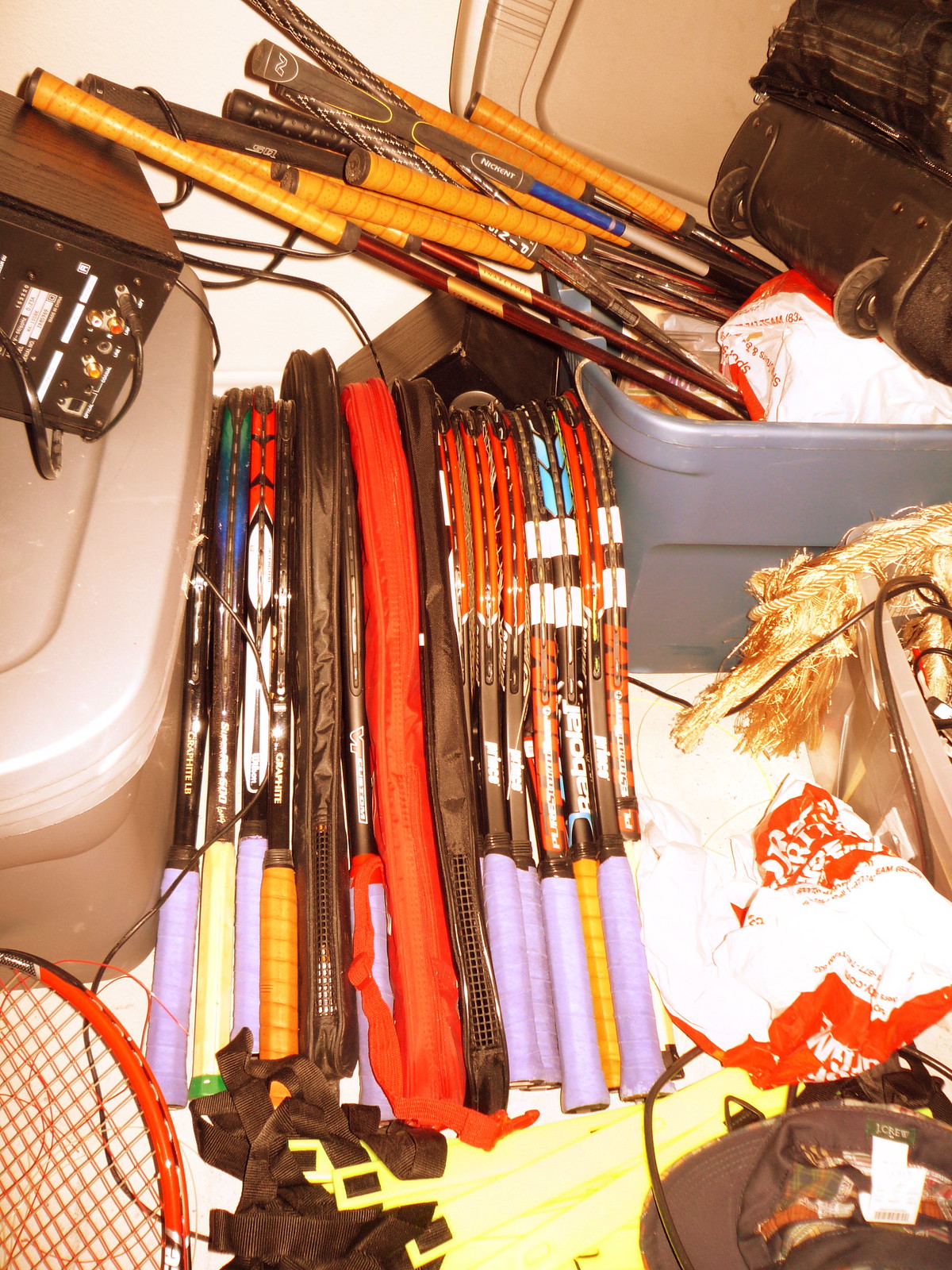The digital image captures a cluttered storage or junk room, possibly a garage, with an assortment of sporting equipment and miscellaneous items. On the left, a black electronic device with fake brown wood paneling and a protruding black cable is notable, sitting on top of a gray Rubbermaid container. To its right, wedged between this and a blue Rubbermaid container, is an array of approximately twelve tennis rackets with various colored handles, including black, blue, red, and brown, some in brown or black cases. The blue container holds what appears to be old golf clubs, identifiable by their brown leather-wrapped handles, and a black rolling bag is situated on top. Beneath the bag are tan-colored items and a white plastic bag with red markings and unreadable white font. The bottom right corner features a gray bucket, while the bottom left corner houses an old-style brown tennis racket. The room appears disorganized, with a yellowish tinge hinting at the use of a flash to capture the chaotic scene.